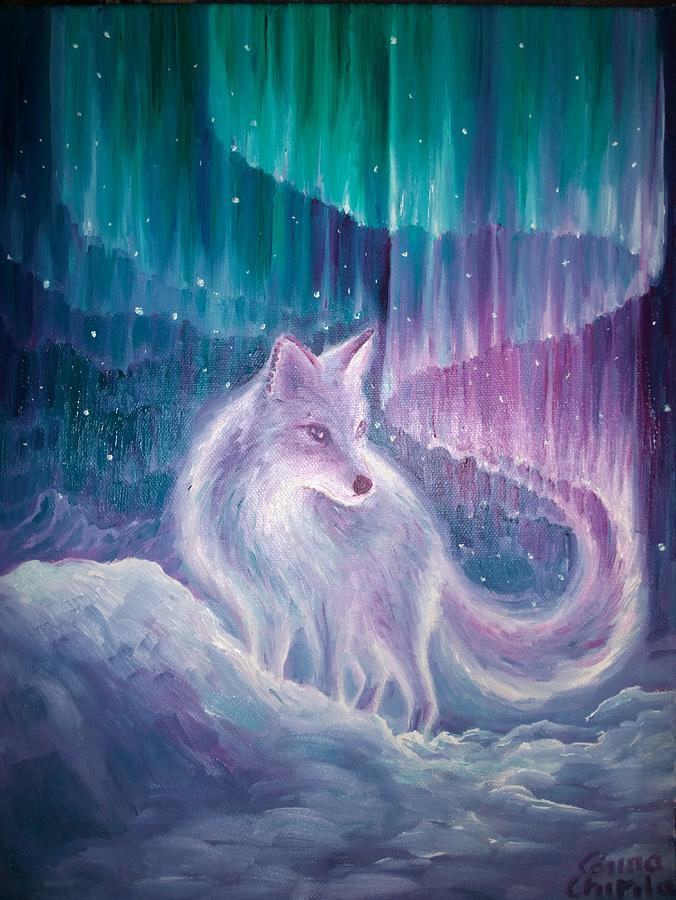In this vibrant and detailed hand-drawn painting, an ethereal arctic fox, rendered in a white hue with delicate touches of pink, purple, and teal, stands majestically in a snowy landscape. The fox, which also resembles a wolf, features distinctive yellowish eyes, a black nose, and black-edged ears. Its long, flowing tail seems to magically transform into swirling streaks of light that fade into an aurora borealis above. This northern light effect is composed of enchanting shades of light teal, deep blue, turquoise, pink, and white, with stars scattered throughout the background, evoking a mystical atmosphere. The fox stands on a hill of packed snow, with additional hand-drawn layers of snow beneath. The artistic style is more whimsical and slightly abstract, blending painting and possibly pastel techniques to create a dreamy effect. The image captures the fox looking slightly off to the right, engaging the viewer with its almost spiritual presence. At the bottom right corner of the image, the artist's signature is present, but it is not legible.